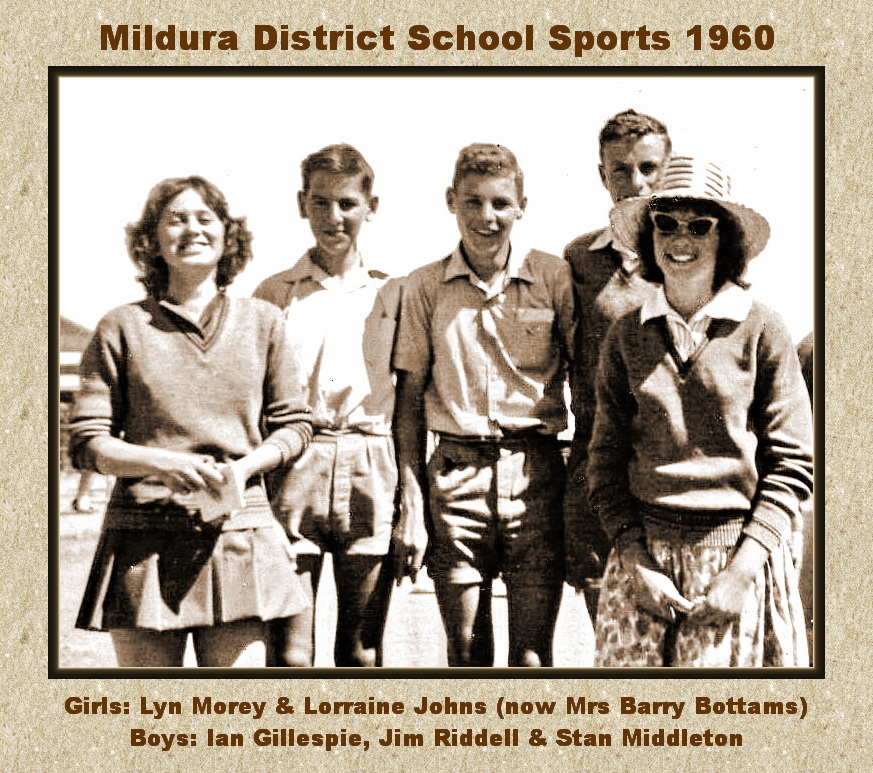This black and white, slightly sepia-toned vintage photograph captures a group of five teenagers from the Mildura District School Sports event in 1960. The image features two young women and three young men, all dressed in period-appropriate attire. The woman on the left is smiling and holding an envelope or a similar item in her hand. She is dressed in a short skirt, reminiscent of a school uniform, paired with a V-neck sweater over a collared shirt. The woman on the right is adorned with a V-neck sweater as well, but instead of a short skirt, she sports a polka-dotted skirt, a straw hat, and sunglasses.

Among the young men, the one on the far left and the one in the middle are both dressed in button-up shirts and shorts, with the middle one smiling broadly. The third young man, positioned slightly behind the woman on the right, is partially obscured. The surrounding gray border frames the photograph nicely, with text at the top reading "Mildura District School Sports, 1960." Listed at the bottom are the names of the individuals: "Girls: Lynn Morney and Lorraine Johns, now Mrs. Berry Bottoms; Boys: Ian Gipsbill, Jim Riddle, and Stan Middleton." The background of the photo subtly features what seems to be dirt, sand, or corkboard, adding to its nostalgic charm.